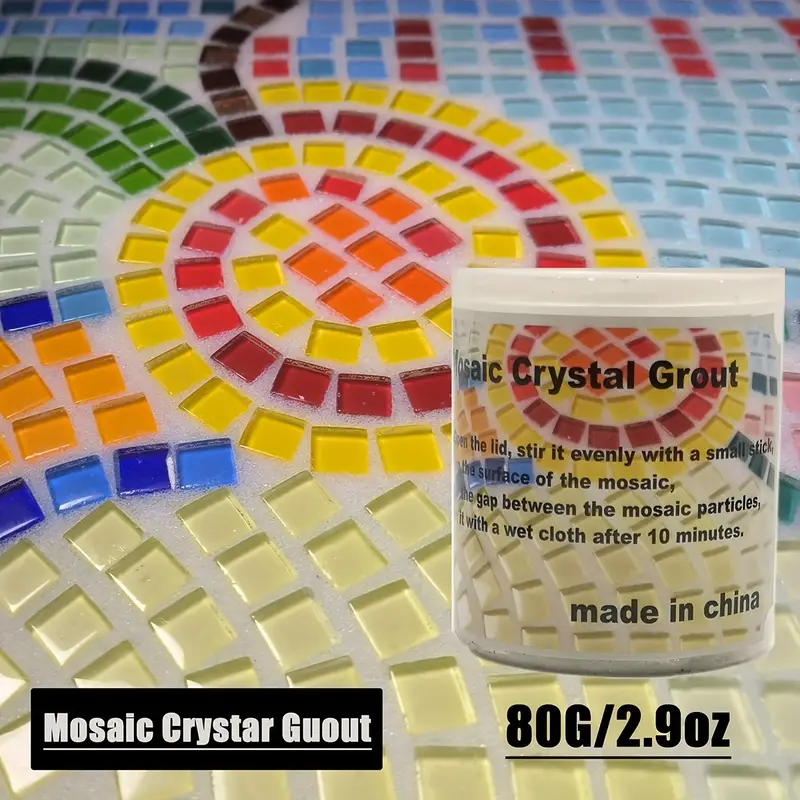The advertisement showcases a 2.9-ounce jar of Mosaic Crystal Grout prominently positioned towards the center-right. The jar, featuring a white lid, displays the label "Mosaic Crystal Grout" in bold text. Instructions on the jar include: "stir evenly with a small stick, fill the gap between mosaic particles, clean with a wet cloth after 10 minutes." Additionally, the jar indicates the product is "Made in China." The background features a striking mosaic made of various colored crystals shaped into small squares. These vibrant tiles form intricate patterns, including a central spiral composed of black tiles interspersed with yellow, red, and orange hues, while other sections include light blue, red, green, beige, and cream-colored tiles. This mosaic design echoes on the jar, creating a cohesive visual theme. The bottom of the image contains additional product details, including "ADG/2.9OZ" in black text on the bottom right and "Mosaic Crystal Grout" in a black rectangle with white letters on the bottom left.